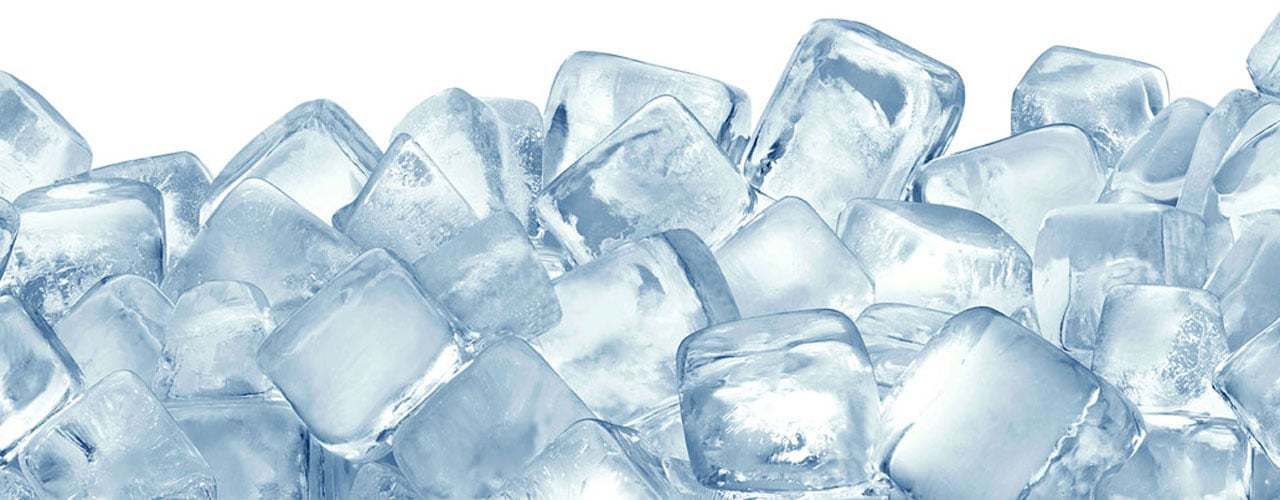The image displays a horizontally-oriented, realistic painting with a white background, showcasing a pile of ice cubes stacked over each other, occupying three-fourths of the frame. The ice cubes feature a dominant bluish tone with teal and dark blue shades, intricate silver reflections, and white highlights that indicate light interplay. The cubes, while predominantly square in shape, have jagged, rough, and slightly rounded edges due to melting. The arrangement looks like a cluster with some gaps between the cubes, enhancing the three-dimensional, layered depth of the scene.